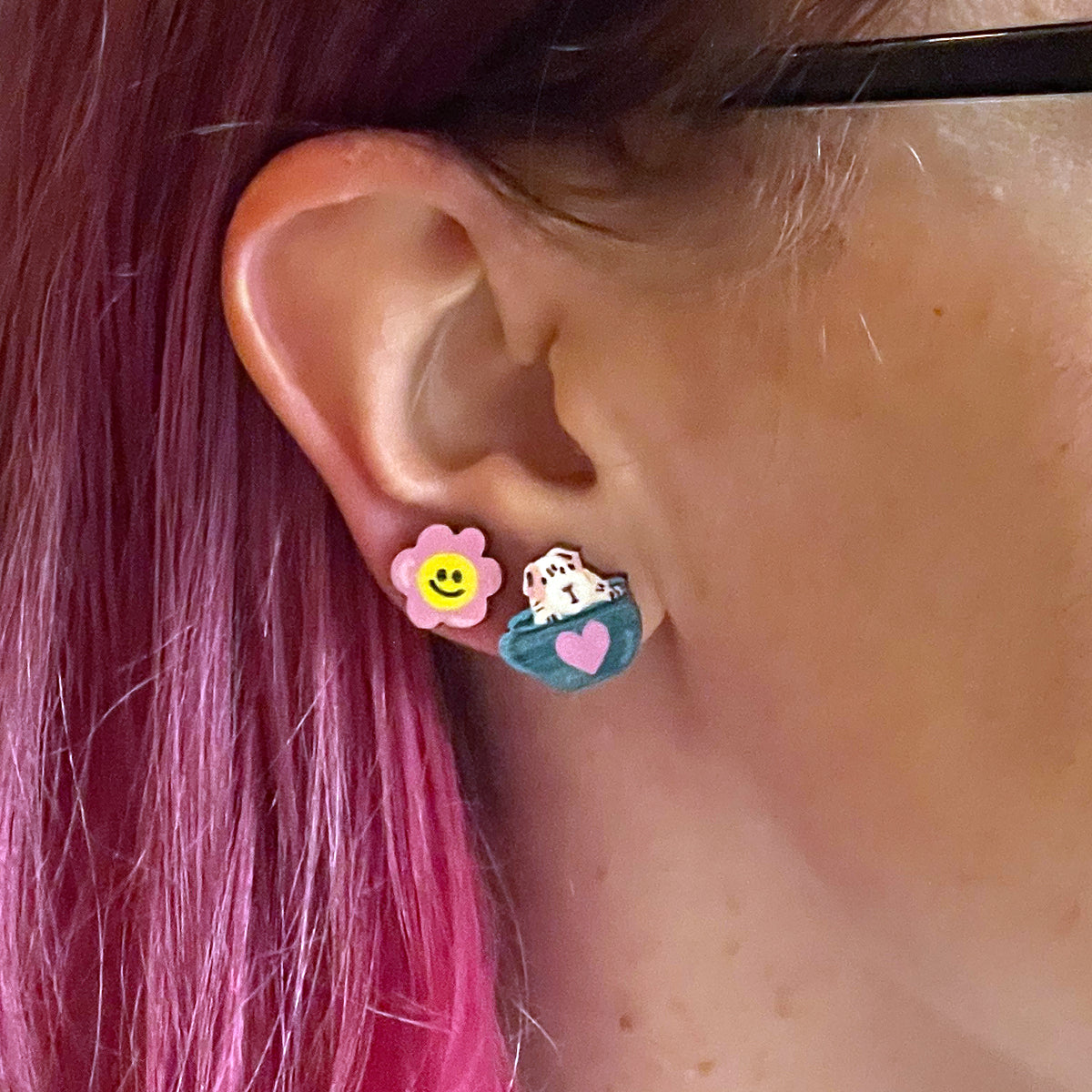A detailed close-up photograph captures the right side of a person's face, prominently displaying their right ear adorned with two distinctive earrings. The person has long, vibrant hot pink hair neatly tucked behind the ear, and their skin is white with some visible blemishes. The upper part of the photo reveals the black frames of eyeglasses extending toward the ear. The earlobe on the ear features homemade earrings: the first earring to the right is a blue cup with a pink heart, out of which a small rodent, possibly a guinea pig or a dog with white and pink accentuated features, appears to emerge. To the left of this earring is another one designed as a pink flower with a yellow center, sporting a black smiley face. The orientation of the face is towards the right, showing a hint of the cheek and neck, enveloped by the shiny pink hair cascading downwards.